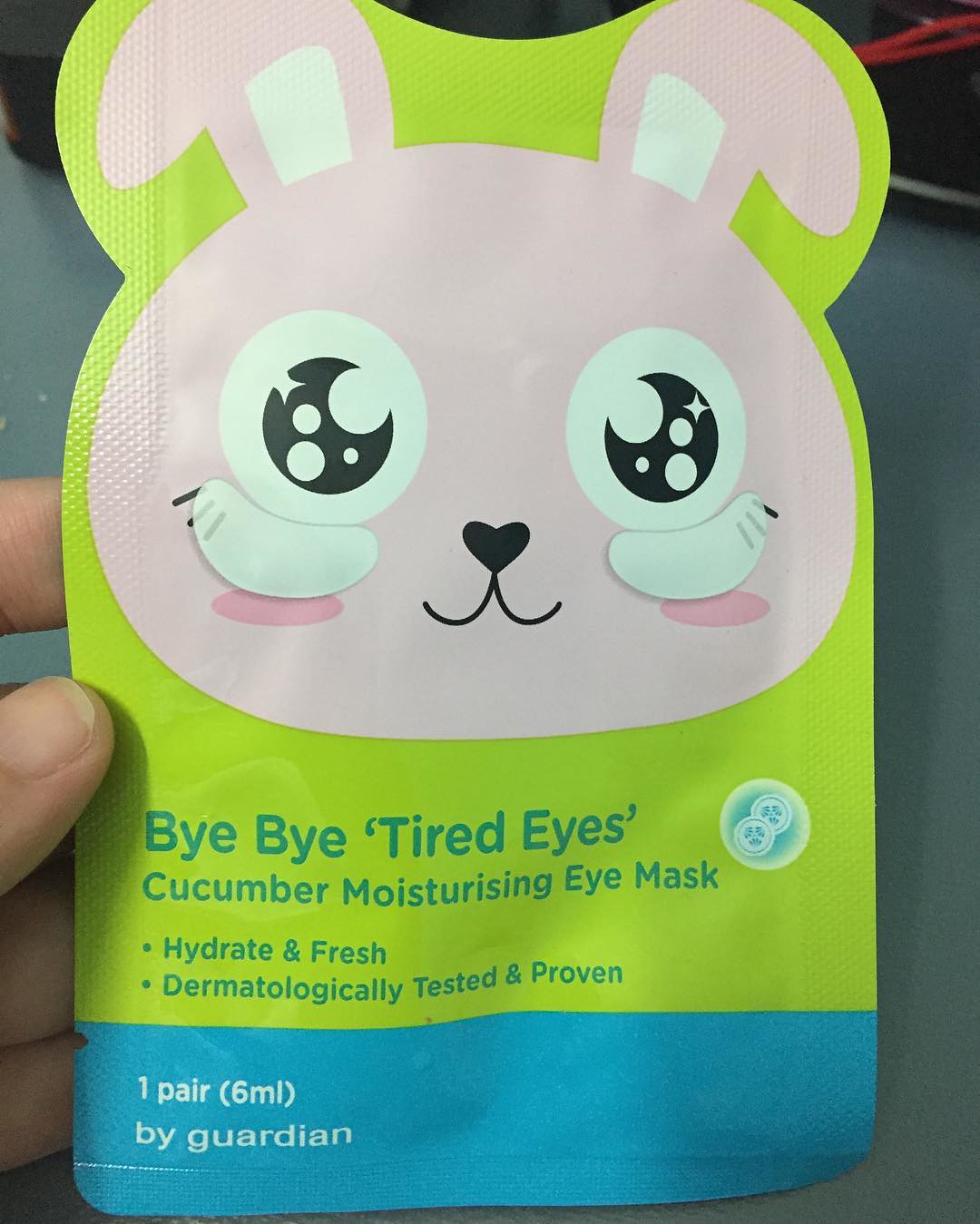The image depicts a close-up of someone's hand holding a packaging for a cucumber moisturizing eye mask by Guardian. The package features a cute, pink cartoon bunny with big, white, doe-like eyes showcasing crescent-shaped pupils filled with stars and circles. The bunny has white inner ears, rosy cheeks, a heart-shaped nose, and a charming smile accented by three lines extending from the sides of its face. Notably, there are two white patches under the bunny's eyes, reinforcing the mask's purpose. Framed by a green border with a lower blue section, the text on the package reads, "Bye-bye tired eyes," in blue font over the green backdrop. Further down in white text against the blue background, it states, "Cucumber Moisturizing Eye Mask," followed by bullet points highlighting "Hydrate and Fresh" and "Dermatologically Tested and Proven." At the bottom, it specifies the contents as "One Pair, 6ml," and mentions the brand Guardian. In the background, a gray sneaker with red shoelaces is visible.